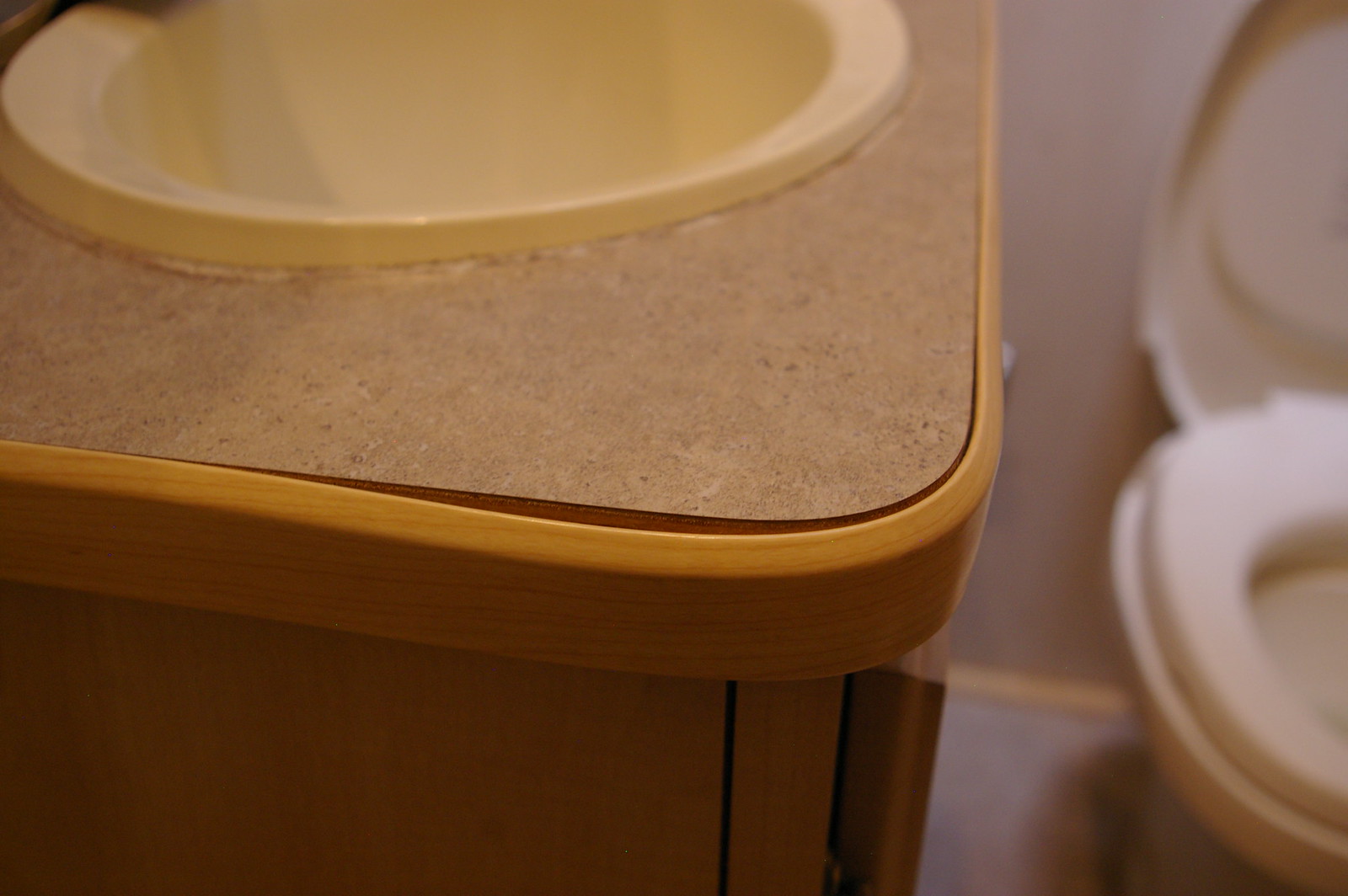A detailed close-up photograph of a bathroom counter and sink area. The left two-thirds of the image are in sharp focus, highlighting a beige, slightly marble-patterned Formica countertop with an ivory-colored, oval-shaped sink basin. The upper portion of the sink is cut off, concealing the faucet. The caulking around the sink is uneven and patchy. The rounded edge of the counter features a light-colored wooden trim with a beveled edge, which does not align perfectly, revealing a gap at the corner. Below the counter, a vertical wood panel of a similar hue is present, with a closed cabinet door visible on the right side. The right one-third of the photograph fades into an out-of-focus background, showing half of a white toilet with a raised lid and a lowered seat. The toilet's minimalistic design lacks a large tank or cistern, and the wall behind it is beige with a light wood baseboard and a gray floor.